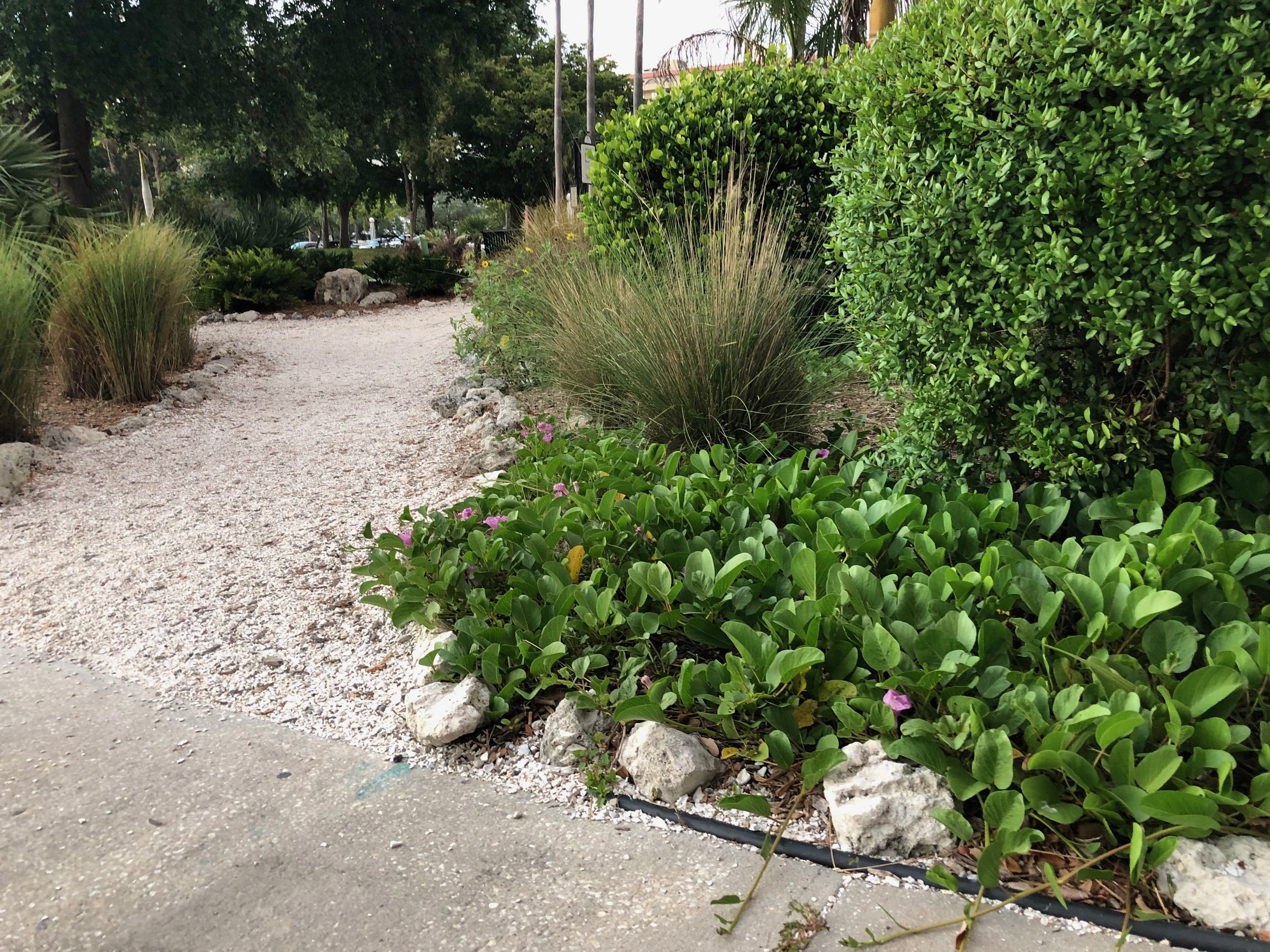The photograph features a serene garden scene with a concrete sidewalk running diagonally from the lower left to the lower right. Adjacent to this sidewalk is a white gravel path that bisects the garden space. On the left side of the path, tall, green, whisker-like plants extend three to four feet high, backed by dense shrubbery and taller trees creating an abundant green canopy. To the right of the path, a small garden area flourishes with greenery. A row of five small white rocks align with the edge of the sidewalk, demarcating a patch filled with low-growing, succulent, green leaves. This leads to another whisker-like plant near the center of the scene, surrounded by lush green bushes. In the upper right, a neatly manicured, ball-shaped bush adds a touch of formality. Beyond this verdant setting, a section of a roof is visible, peeking through the foliage near the top center of the image, and distant elements like flagpoles, trees with green leaves, and possibly a parking lot can be seen faintly in the background. The overall ambiance suggests a location possibly in the southwestern United States or California, and the entire scene is awash in lush, natural greenery.